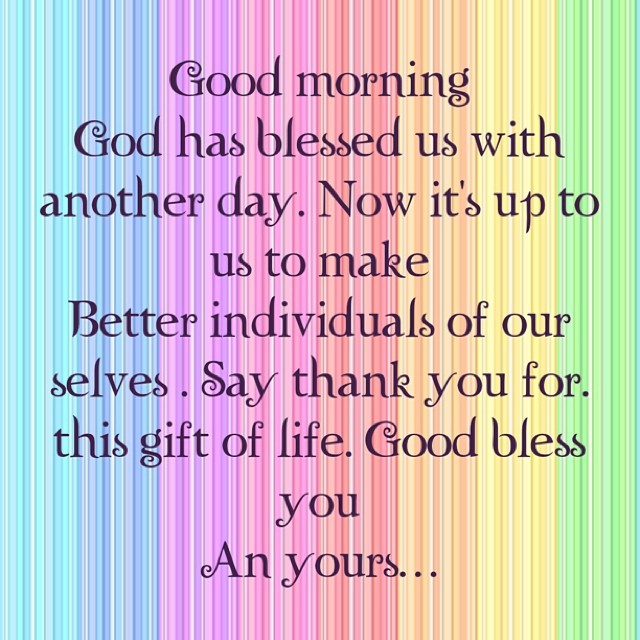This digitally generated image features a vibrant, multi-colored background comprised of vertical stripes in various shades of blue, teal, purple, pink, red, orange, yellow, and green. Superimposed over this colorful backdrop is a motivational message in black, creatively-styled text. The uplifting quote reads: "Good morning. God has blessed us with another day. Now it's up to us to make better individuals of ourselves. Say thank you for this gift of life. God bless you and yours." Despite a minor typographical error in the phrase "God bless," where it appears as "Good bless," the message remains clear and encouraging.